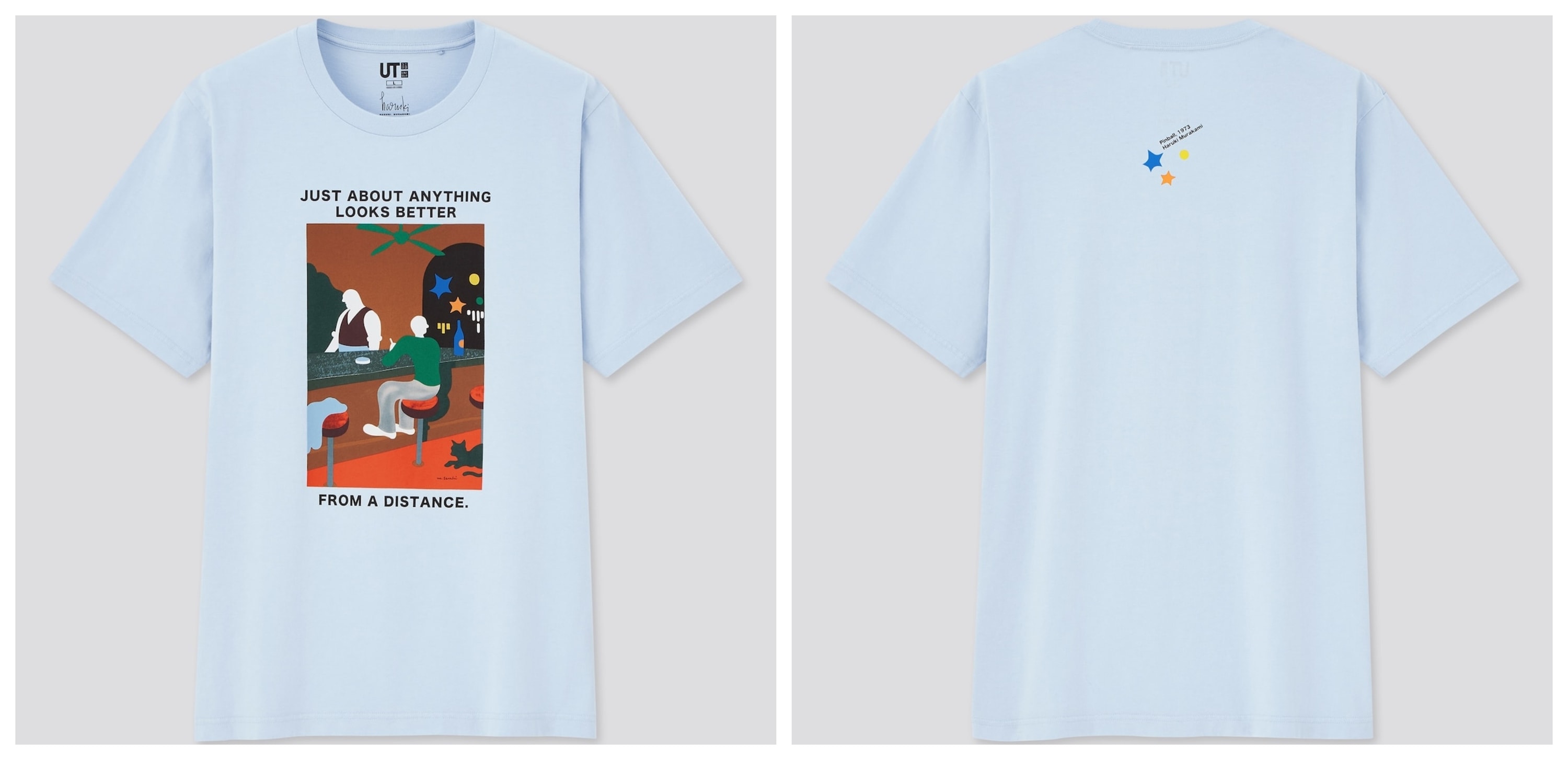This dual-image showcases both the front and back views of a white short-sleeve crew neck shirt. The first image presents the front side of the shirt. It features a rounded, slightly thick collar that sets apart the neck area from the rest of the garment. The sleeves are subtly tucked underneath and do not protrude outward. 

On the front, the shirt displays the letters "UT" at the top, followed by some additional text that appears to be part of a tag. Prominently, there is an illustration resembling computer-generated clip art, depicting a scene in a bar. The illustration shows a character wearing a green shirt, gray pants, and white shoes, seated on an orange bar stool. To the right stands the bartender, with a ceiling fan above and several stars scattered on the right side of the image. The caption within the illustration reads, "just about everything looks better."

The back view of the shirt is simpler, featuring a small clip art design consisting of two stars and one circle, with some text above the illustration. Specifically, it includes one large blue star, a smaller yellow star, and a yellow dot.